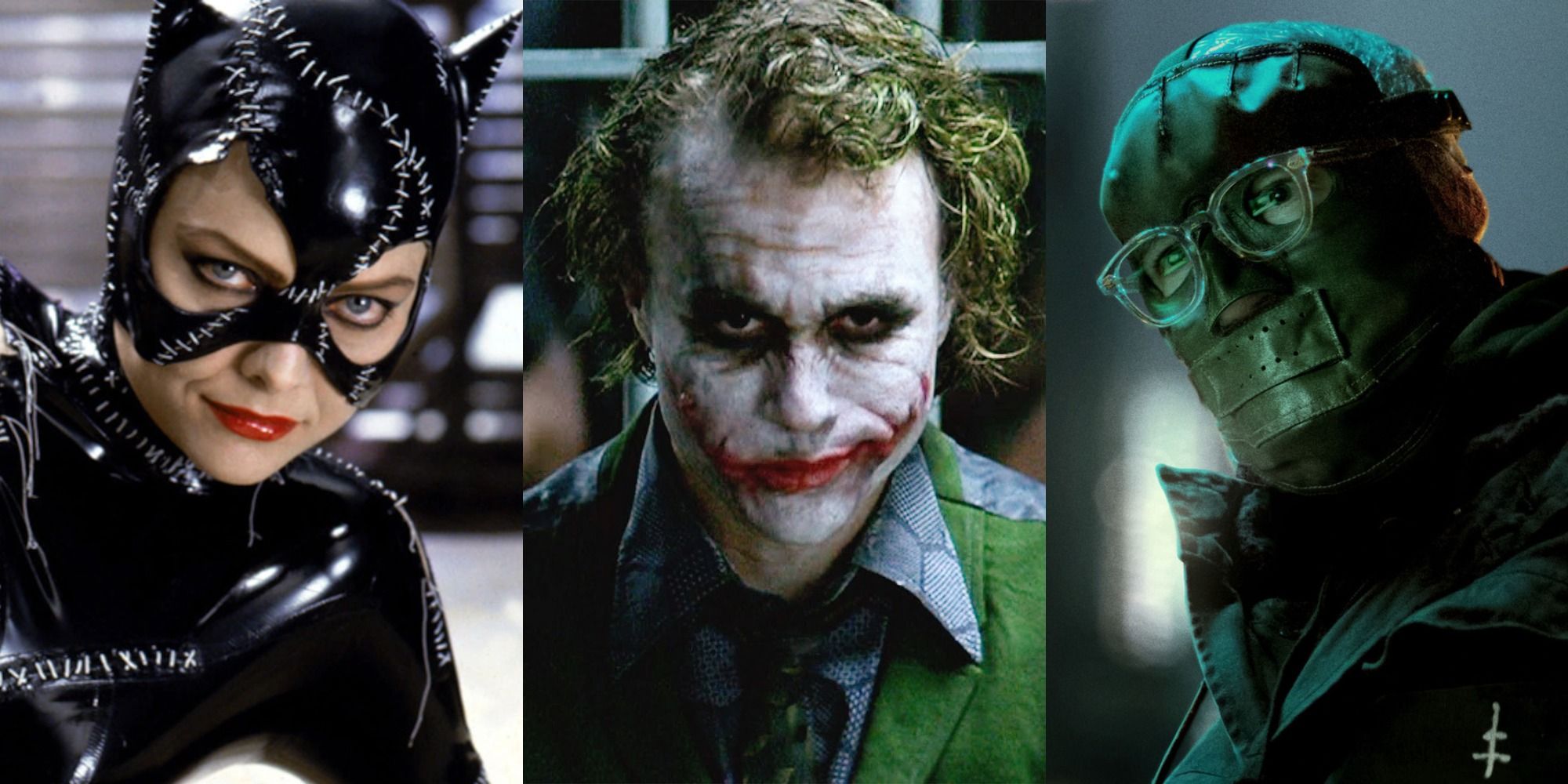The photograph is a triptych showcasing three iconic characters from the Batman series, each portrayed by notable actors. On the far left, we see Michelle Pfeiffer as Catwoman, donning a black shiny latex outfit with a stitched appearance, complete with cat ears and red lipstick, looking directly at the camera. The center image features the Joker from Christopher Nolan's "The Dark Knight," characterized by his smeared white face makeup, dirty green hair, exaggerated red lips reaching to his cheeks, black eye makeup, and a mismatched suit of green and light purple hues. To the right is Paul Dano as the Riddler from "The Batman," wearing a dark green jacket with a conspicuous white symbol that appears to be an upside-down cross with an extra line. His face is obscured by a green leather mask, except for his eyes which are covered by thick, clear glasses like safety goggles.